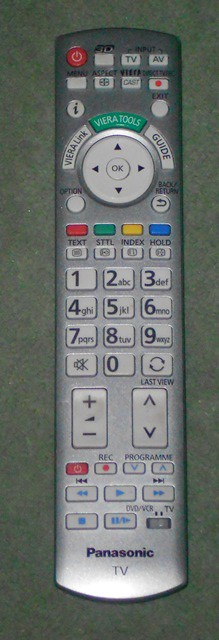The image is a close-up photograph of a slender, tall remote control for a Panasonic TV, resting on a dark hunter-green background with a marbled texture. The remote itself is an elegant, steely, silver-gray color, featuring a variety of multi-colored buttons. At the very top left, there is a prominent red power button. Just below it, there is a 3D button and several additional buttons including Input TV/AV, Menu, Aspect, and Direct TV Exit, which is marked with a small red spot.

The middle section of the remote showcases a white circular pad surrounded by directional arrows (up, left, right, down) and an OK button in the center. Above this pad are three semi-circular buttons labeled Viera Link (in white), Viera Tools (green), and Guide (white). On the left, a button is labeled Option, and on the right, there's a button that says Back/Return with an arrow pointing to the left.

Below the circular pad are several function buttons: a red Text button, a green STTL button, a yellow Index button, and a blue Hold button. Further down, there is a numeric keypad featuring numbers 0 through 9, a mute icon at the bottom left, and a last view icon at the bottom right.

Towards the bottom section, there are volume controls and buttons for recording programs, alongside various playback controls including Play, Pause, Fast-forward, Rewind, and Stop. The remote also includes controls for DVD, VCR, and TV devices. Finally, at the very bottom, the Panasonic logo is displayed in black text, along with the word "TV" underneath it.